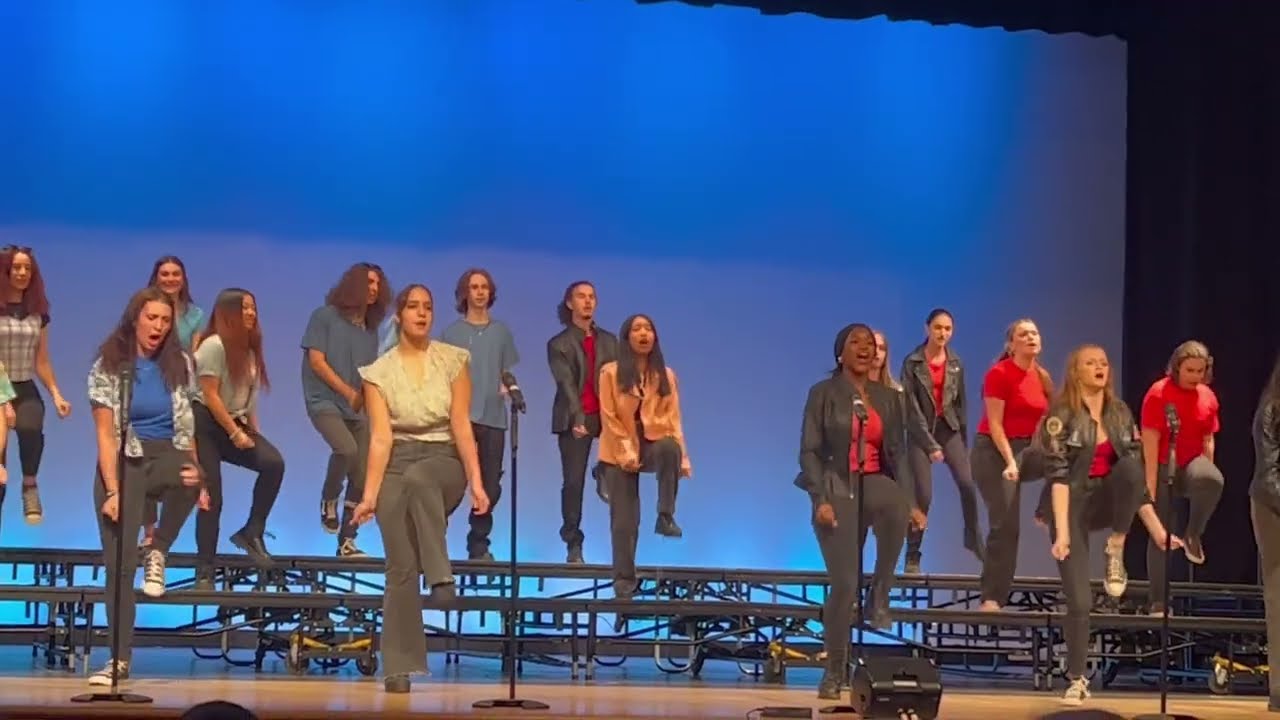In this detailed image, we observe a group of seventeen women standing on a stage, appearing to be performing a choreographed routine. All of them are in black pants, and while the group on the right side also wears red t-shirts, the left side showcases a variety of colorful shirts in pink, white, green, and blue. The women on the far left edge notably have long hair. Three individuals wear black jackets. The stage features a tiered wooden platform or bleachers occupying the lower third, with five women standing in front of it beside four prominently positioned microphone stands. The backdrop is illuminated with ambient blue light projected from both the top and bottom, adding depth to the scene. The setting appears to be an indoor performance center with a wooden floor, but no text is visible on the image. The arrangement and attire suggest a concert or choir performance, with the women raising their left legs in unison, enhancing the impression of synchronized movement.